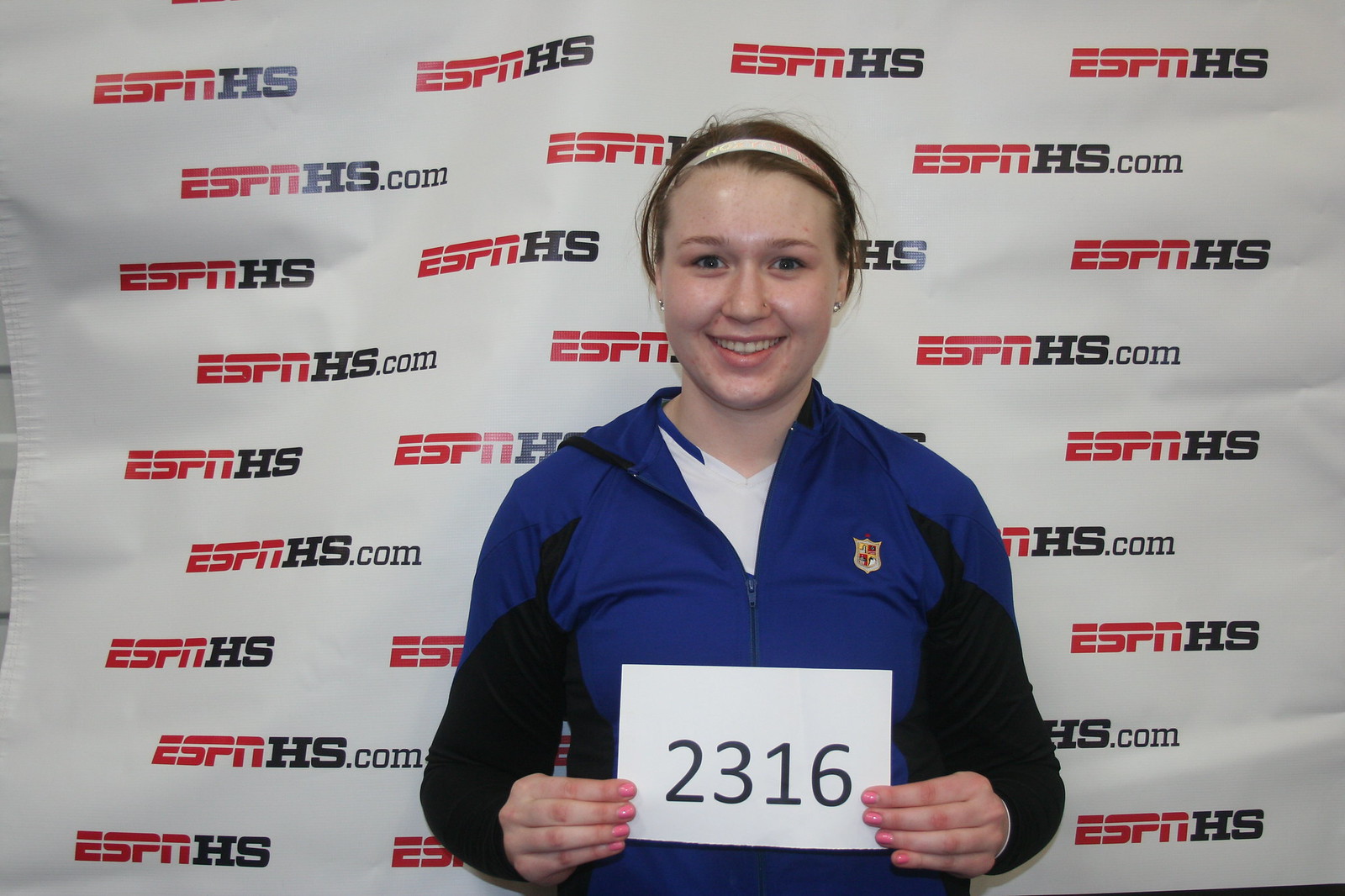In the photograph, a young girl, possibly around 12 or 13 years old, stands confidently while holding a white sheet of paper with the number "2316" printed in bold black letters. She is smiling warmly, with a look of determination and joy on her face. Her short brown hair is accented with a pink hairband, and her nails are painted a matching pink. She is dressed in a blue and black sports jacket, which is slightly unzipped to reveal a white and blue v-neck shirt underneath. The jacket features some type of crest on the right breast. Behind her is a white backdrop decorated with a repetitive logo featuring "ESPNHS" in red and black, and "ESPNHS.com."